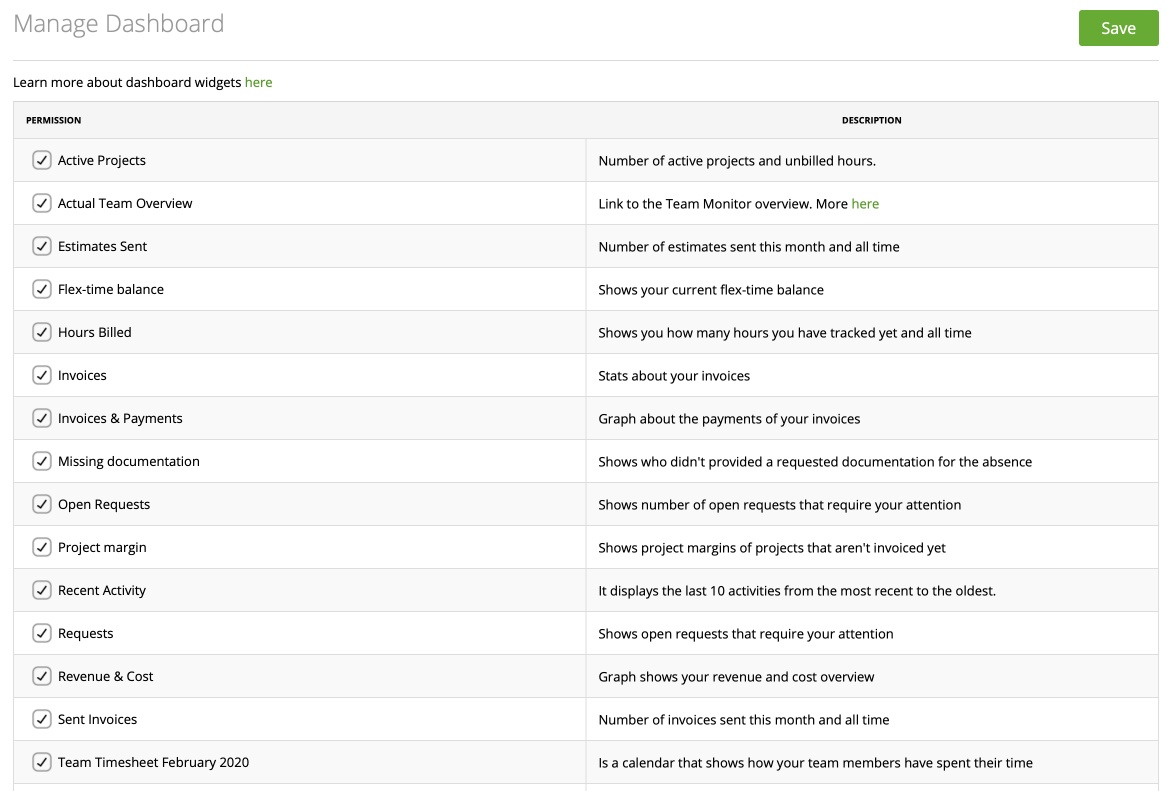**Dashboard Overview: February 2020**

This comprehensive dashboard provides a detailed view of various project management metrics and team activities. Key features include:

- **Permission and Active Projects:** Displays the number of current projects and gives an overview of team activities and permissions.
- **Estimates Sent:** Shows the number and details of estimates sent both this month and historically.
- **Flex Time Balance:** Indicates your current balance of flex time.
- **Hours Billed:** Tracks the hours billed to clients.
- **Invoices and Payments:** Provides statistics about your invoices and graphs illustrating payment statuses.
- **Missing Documentation:** Identifies team members who have not submitted required documentation for absences.
- **Open Requests:** Lists open requests that need your attention.
- **Project Margin:** Displays margin statistics for projects not yet invoiced.
- **Recent Activity:** Shows the last 10 activities in chronological order from the most recent to the oldest.
- **Revenue and Cost:** Offers a graphical overview of revenue and costs.
- **Sent Invoices:** Keeps track of all invoices sent this month and over time.
- **Team Timesheet:** Calendar view showing how team members have allocated their time.
- **Current Free Time Balance:** Indicates how many hours you have tracked so far.
- **Team Monitor Overview:** Provides a link to monitor team activities in detail.
- **Stats and Graphs:** Includes detailed statistics and graphs for deeper insights into various metrics.

Use this dashboard to manage and save your projects, learn more about the widgets available, and keep track of the different aspects of your team's performance and project statuses.